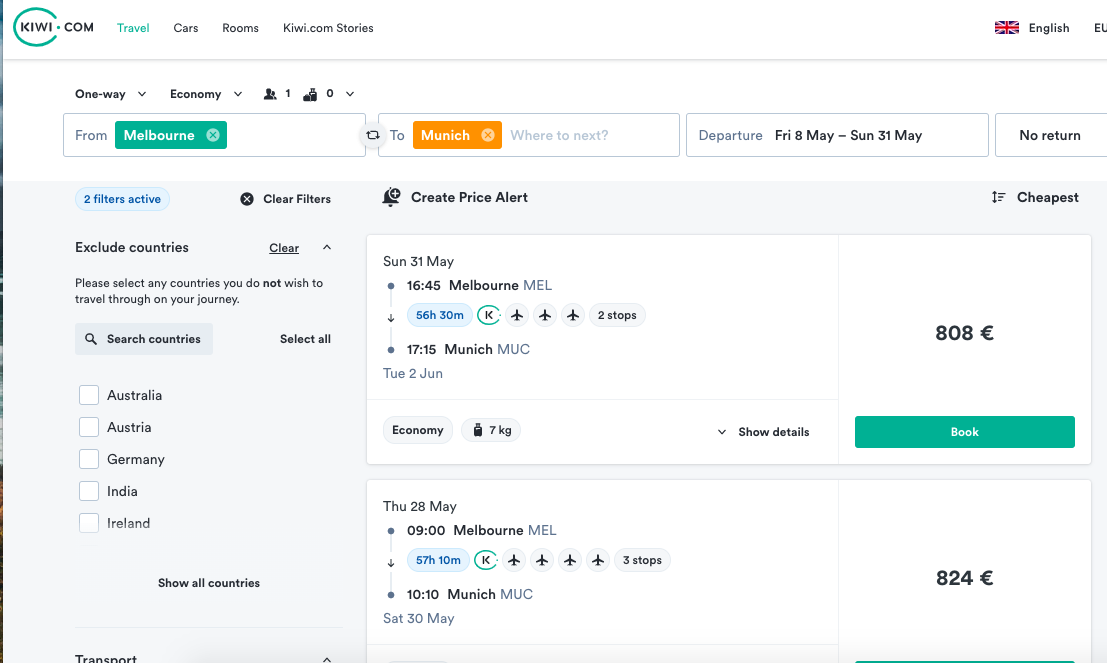This screenshot captures the homepage of a travel website, Kiwi.com. In the top-left corner, the logo features the word "Kiwi" highlighted within a green oval, and a green dot completes the ".com" suffix. The navigation menu offers several options: "Travel," "Cars," "Rooms," and "Kiwi.com stories."

On the far right side of the menu bar, there's an icon of the British flag, indicating the language selection is set to English. A thin gray line separates the navigation menu from the content below.

Towards the left section of the page, there are multiple dropdown menus labeled "One way," "Economy," and "One person," along with an icon suggesting zero luggage items. Below these options, departure information is provided: the journey is from Melbourne (highlighted in a green box) to Munich (highlighted in an orange box). The departure date is set for Friday, May 8th, and the return date is specified as Sunday, May 31st.